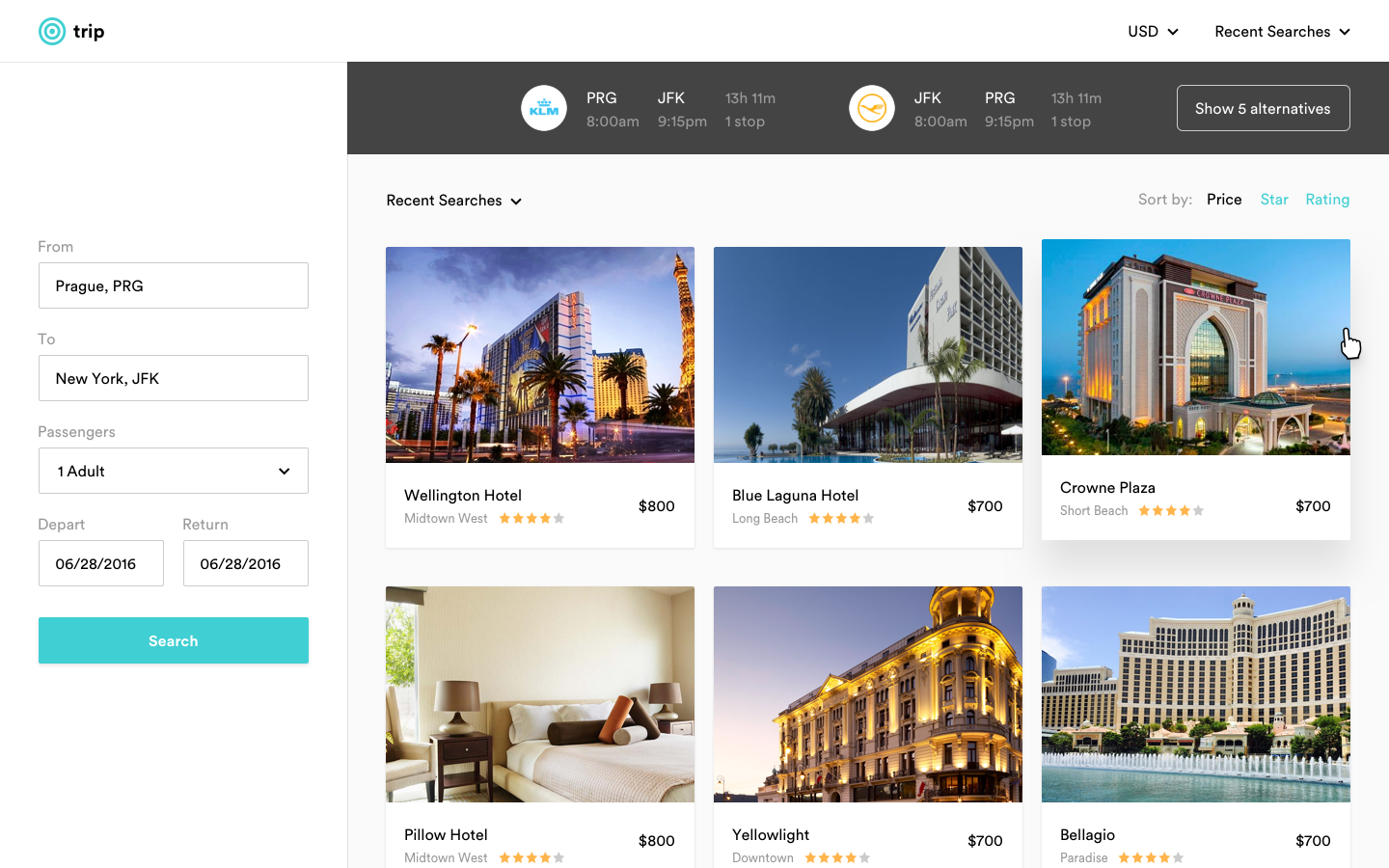Here is the cleaned-up and detailed caption:

---

This image is a screenshot from a computer screen showcasing a travel booking website. In the top left corner, a teal bullseye icon consisting of a dot and two concentric circles is displayed next to the word "Trip" in black text. Below this, a gray line extends horizontally across the screen.

On the left-hand side of the screen, which has a white background, several sections are visible:
1. Below the "Trip" label, the word "From" is written in gray, followed by a gray outline box containing the black text "PRG."
2. Underneath, the destination is indicated with "To New York, JFK" in black text.
3. The next line specifies the passengers as "One adult" with a drop-down arrow.
4. The departure date is shown as "06-28-2016" and to the right, the return date is also "06-28-2016."
5. A teal bar labeled "Search" in white text is positioned below these details.

On the right-hand side, also with a white background, the following elements are visible:
1. The text "USD" in black with a drop-down arrow.
2. To the right, another drop-down arrow labeled "Recent Searches."

The main part of the screen features a black box extending from the left side to the right. This box includes an icon with a white circle containing teal text that says "KLM" and an image resembling a sombrero. Black text within this part indicates "PRG 8 AM" in gray, followed by "JFK 9-15 PM" in white. The duration "13H11M" and "one stop" are noted beneath. Another flight option is listed similarly with a white circle and an orange icon that could be an orange foot or bird, detailing "JFK 8 AM" and "PRG 9-15 PM," also with a duration of "13H11M" and "one stop." Below, a gray outline box in white reads "Show five alternatives."

Continuing downward, a section with a gray background displays:
- "Recent Searches" in black with a drop-down arrow
- "Sort by: Price" in gray, "Rating" in teal, and an asterisk

A series of hotel images and descriptions are also shown:
1. **Wellington Hotel:** A high-rise located in Midtown West, featuring an adjacent high-rise, columns to the left, palm trees, a street light, and a structure resembling the Eiffel Tower in the background. Rated four orange stars and one gray star, priced at $800.
2. **Blue Laguna Hotel:** Located in Long Beach, a high-rise with a triangular overhang above the lobby, surrounded by palm trees and the ocean. Rated four stars, priced at $700.
3. **Crown Plaza:** A well-lit high-rise in Short Beach, resembling the Champs-Elysees with lighted indentations on the left side, bordering the ocean and greenery. Features an entrance for luggage drop-off, lit roadways, and ocean views. Rated four stars, priced at $700.
4. **Pillow Hotel:** Located in Midtown West, the image shows a double bed with lamps and nightstands on either side, a chair by a window with a brown shade. The hotel is four stars, priced at $800.
5. **Yellow Light Hotel:** A triangular four-story building with a rounded front and a gazebo-like structure on top, all lit up. Located downtown, it is rated four stars and priced at $700.
6. **Bellagio:** A large concave high-rise in Paradise, accompanied by a shorter building on its left. The foreground features smaller buildings, an entrance, white water fountains, and a pond. Rated four stars, priced at $700.